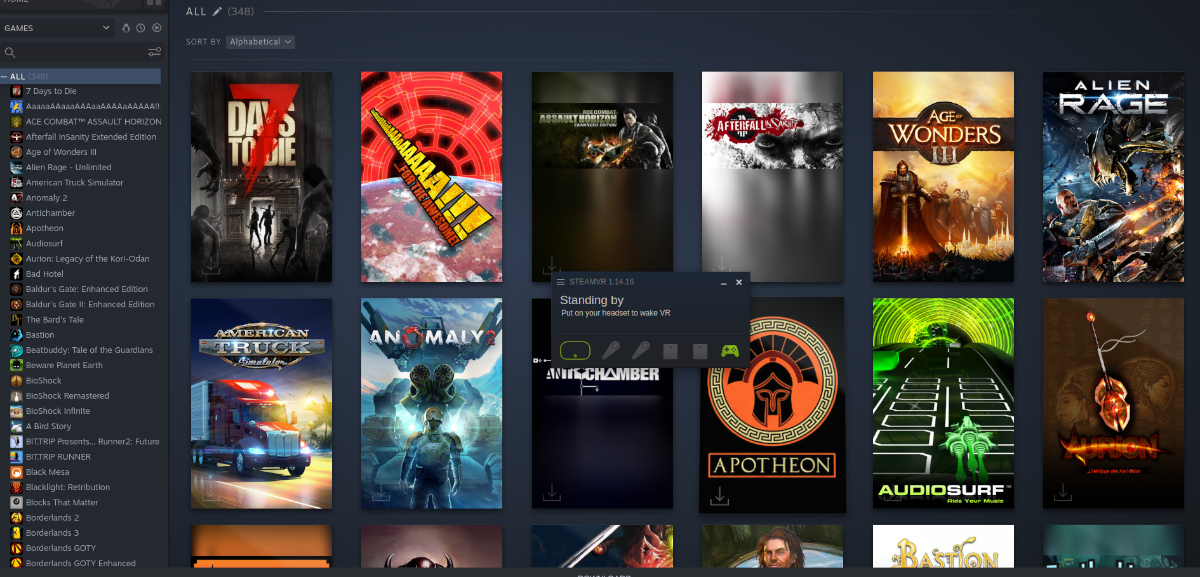Screenshot of a Steam Library Interface Featuring VR Prompt and Game Collection

The image is a screenshot of a gaming library, likely from the popular gaming platform Steam, given the interface layout and design. The screenshot appears slightly cut off with no visible branding, but several notable features can be identified.

On the left side of the screen, there is a search bar specifically for finding games within the user's library. Below this are the visible icons and titles of about 30 games, organized in a vertical list. The total number of games in the user's collection is stated to be 348, although only titles from the first few alphabetical rows are visible. The games listed include popular titles such as "Borderlands," indicating the user's extensive library.

On the right side of the screen, the games are sorted alphabetically and shown in a more detailed list. Visible game titles include "Seven Days to Die," "I," "Afterfall," "Age of Wonders," "Age of Wonders III," "Alien Rage," "American Truck Simulator," "Anomaly," "Antichamber," "Apotheon," "Audiosurf," and "Ariane." Only two rows of game titles are legible before being cut off.

Additionally, there is a pop-up message regarding Steam VR, version 1.14.35. The prompt seems to be instructing the user to put on their VR headset or use VR-related equipment, as indicated by the text "standing by, put on your headset to wake." Below this message are various icons representing VR equipment, including a VR headset, two handheld controllers, two tracking boxes, and a gamepad. The icons for the VR headset and gamepad are highlighted in green, suggesting these items need to be activated or are currently ready for use.

Overall, the image depicts a detailed view of a Steam user's extensive game library, alongside a VR prompt indicating the readiness of the system for a virtual reality experience.